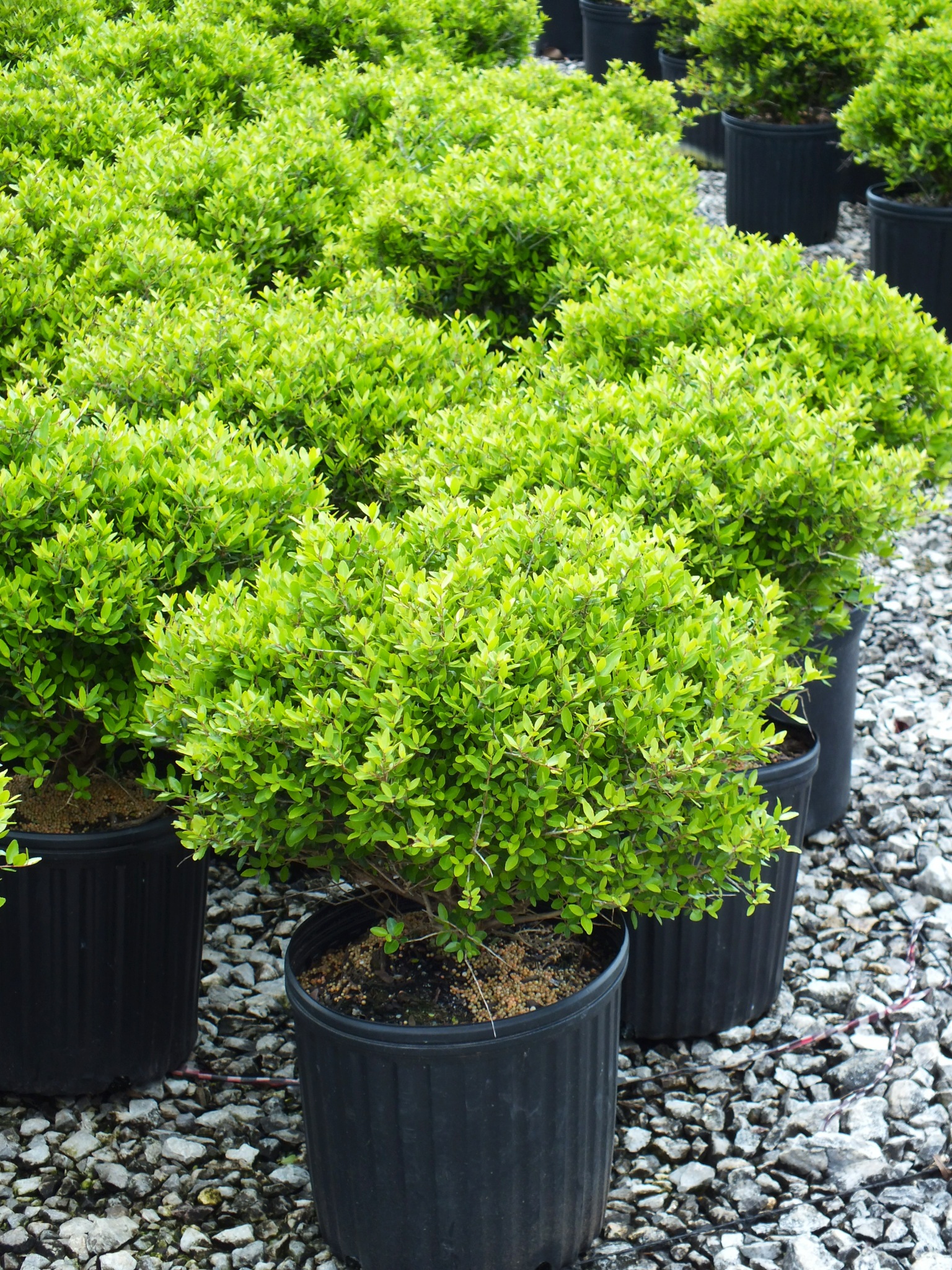This photograph captures a dense grouping of small, vibrant green bushes, all potted in tall, black plastic containers. These pots, filled with rich, dark soil enhanced with plant nutrients, are tightly clustered together, likely indicative of a nursery or garden supply store setting. The backdrop reveals a ground made of grey gravel stones, adding to the neat and organized display. Each bush, identical to the next, sports a bright green hue, reflecting the well-lit, likely daylight conditions despite an overcast sky. This setup suggests the plants are ready for purchase and replanting elsewhere, ideal for creating dense, small-leaved hedges.